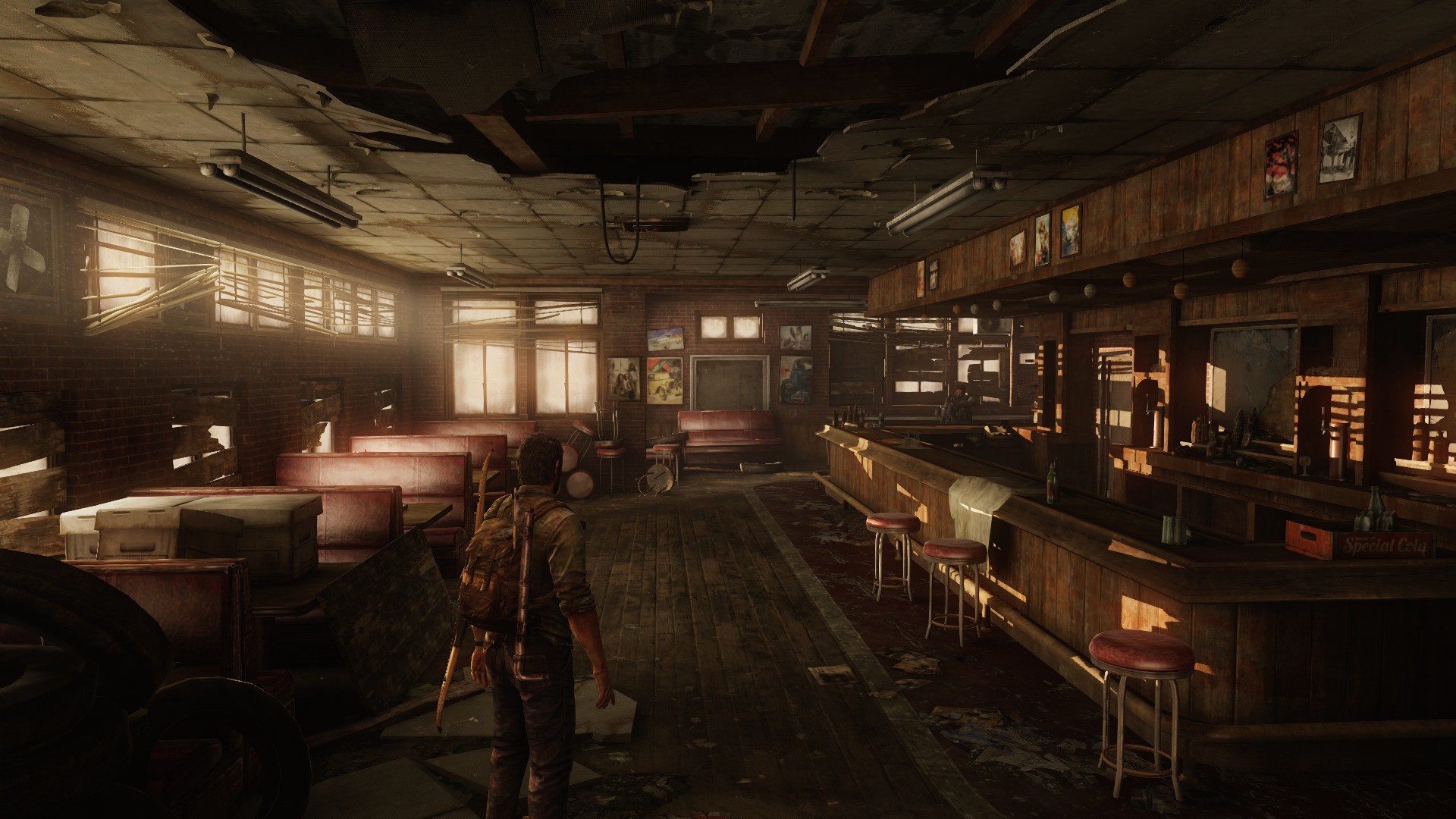This colored illustration, reminiscent of a scene from a video game, captures the interior of a deserted restaurant or bar. The viewer’s perspective is from within, highlighting a solitary figure standing with their back to us. This person, sporting short brown hair, dons a greenish shirt with the sleeves rolled up to the elbows. A green backpack clings to their back, equipped with a long, double-ended weapon. They are casually dressed in jeans and stand on a grimy wooden floor. 

To the right, three small bar stools are aligned with a rustic wooden bar. Light penetrates through a window with broken wood paneling, illuminating the otherwise dingy atmosphere. On the left side, five booths appear neglected, covered in dust, with some serving as makeshift storage for cardboard boxes. Adjacent to these booths, a brick wall supports windows that are boarded up and partially shattered at the top. The blinds, though present, are disordered and displaced, contributing to the scene's overall state of disarray.

Towards the back, a sizable window also features disheveled blinds, amplifying the sense of abandonment. Bar stools are scattered, piled up and overturned against the rear brick wall, further emphasizing the decay and forsakenness of the establishment.